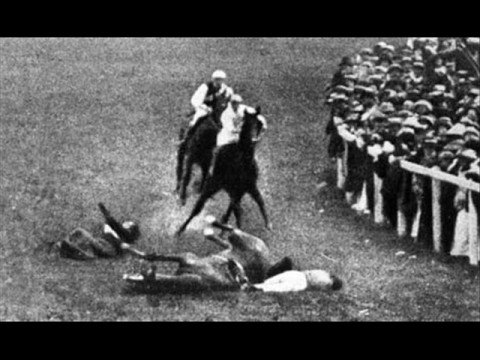This black-and-white photograph, likely over 100 years old and possibly a still from a silent newsreel or film from the early 1900s, captures a dramatic moment during a horse race. The image is grainy and features widescreen black bars typical of old films. The scene unfolds on a racetrack with a curved white fence to the right, behind which a crowd of people is intently watching the race. In the foreground, two jockeys on their horses are attempting to navigate around a catastrophic accident. One horse is lying sideways on the track, its legs splayed out, while two people are seen on the ground, apparently having been dismounted. A jockey lies unconscious to the right of the fallen horse, and a woman is seen with her arm in the air on the left. Dirt and possibly gravel cover the track, adding to the chaotic scene as the surviving horses desperately try to avoid the collision. This moment might even be linked to the historic suffragette movement, known for incidents involving protestors interrupting horse races.